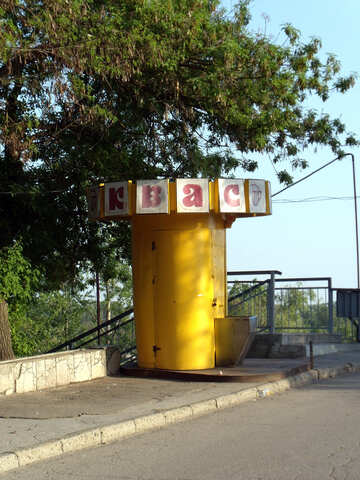The photograph, taken outdoors during the early evening, features a yellow cylinder-shaped structure, possibly an outdoor public restroom given its single-person size, door with hinges, and an attached drinking fountain. On the top edge of this structure, a series of white papers are plastered, each displaying a single red letter: K, B, A, C. These letters are placed around its circumference, likely with additional unseen letters or papers. Adjacent to the letters, there's a drawing of a face or some other illustration. Beside the structure, there is a cylindrical metal trash can or container potentially meant for holding items or collecting coins. The scene includes a descending staircase that leads into a wooded or forested area, with a stone walkway and street visible to the left of the structure.